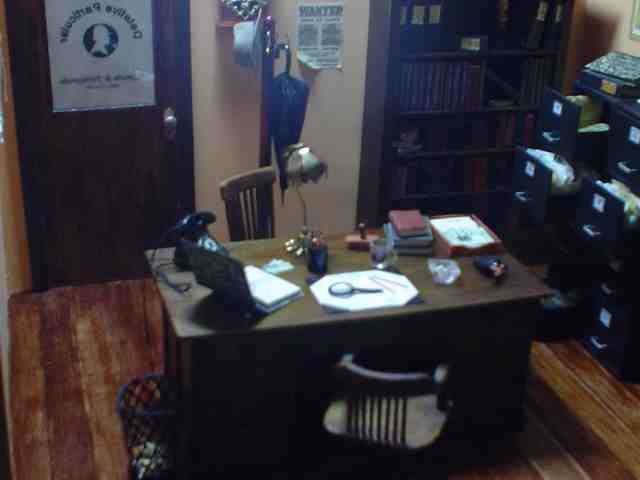The image depicts a well-organized workspace with various elements contributing to a vintage ambiance. A brown desk, placed on reddish-brown flooring, serves as the focal point. To the left of the desk is a brown door featuring a silver handle and frosted white glass. The upper portion of the door is adorned with black lettering and a black circle showcasing a stylized white silhouette of a head.

Adjacent to the door is a brown wall with a sturdy hook. Hanging from this hook are a white hat and a blue umbrella. Mounted alongside is a white piece of paper with black writing. On the desk, a magnifying glass rests on top of a white sheet of paper, while a silver lamp stands prominently in the middle. There are several books placed to the right side of the desk. 

To the top left of the scene is a brown chair, and towards the right, near the edge of the desk, sits an old-fashioned black telephone. An open binder lies on the left side of the desk. Positioned at the bottom left, a blue wastepaper basket is partially visible. In front, there's a small greyish-to-black chair with thin spindles.

To the right, a black bookcase stands, and below it are some grey metal cabinets, all opened, revealing papers inside. Completing the scene, another section of the brown wall is visible at the top right. The detailed assemblage of items creates a nostalgic and meticulously detailed office environment.